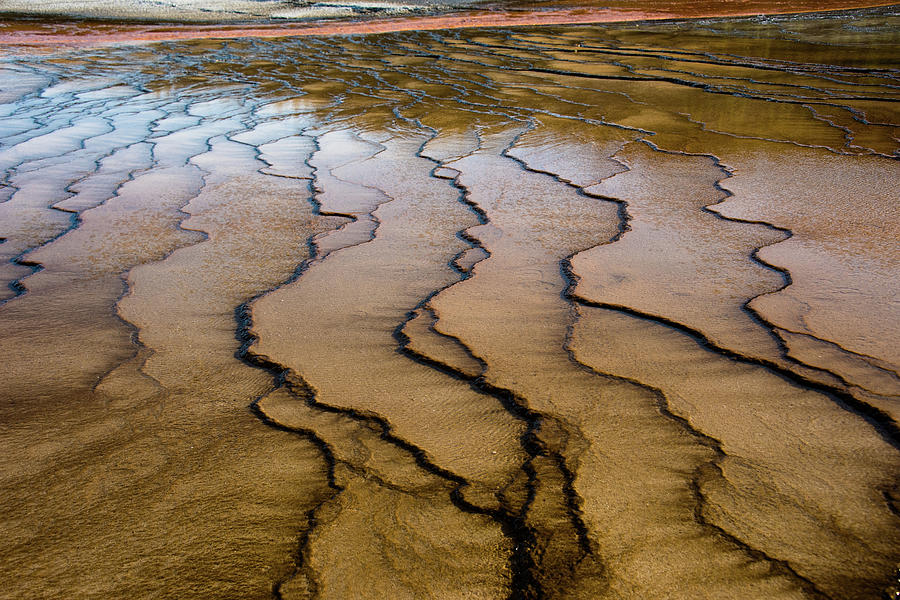The image is a captivating blend of natural and surreal elements, leaving one uncertain if it is an artistic photograph or a meticulously crafted drawing or painting. Dominated by wavy vertical black lines cutting through a predominantly brown and beige background, it evokes both abstraction and realism. The surface appears either wet or covered by a shallow layer of water, hinting at a muddy, possibly sandy terrain. In the background, there's a horizon marked by a thin, red-orange strip that could be a distant landmass or shoreline. The colors are a constrained palette of black, white, various browns, and muted reds, enriching the scene's enigmatic quality. No text or living beings are present, enhancing its mysterious and contemplative nature.